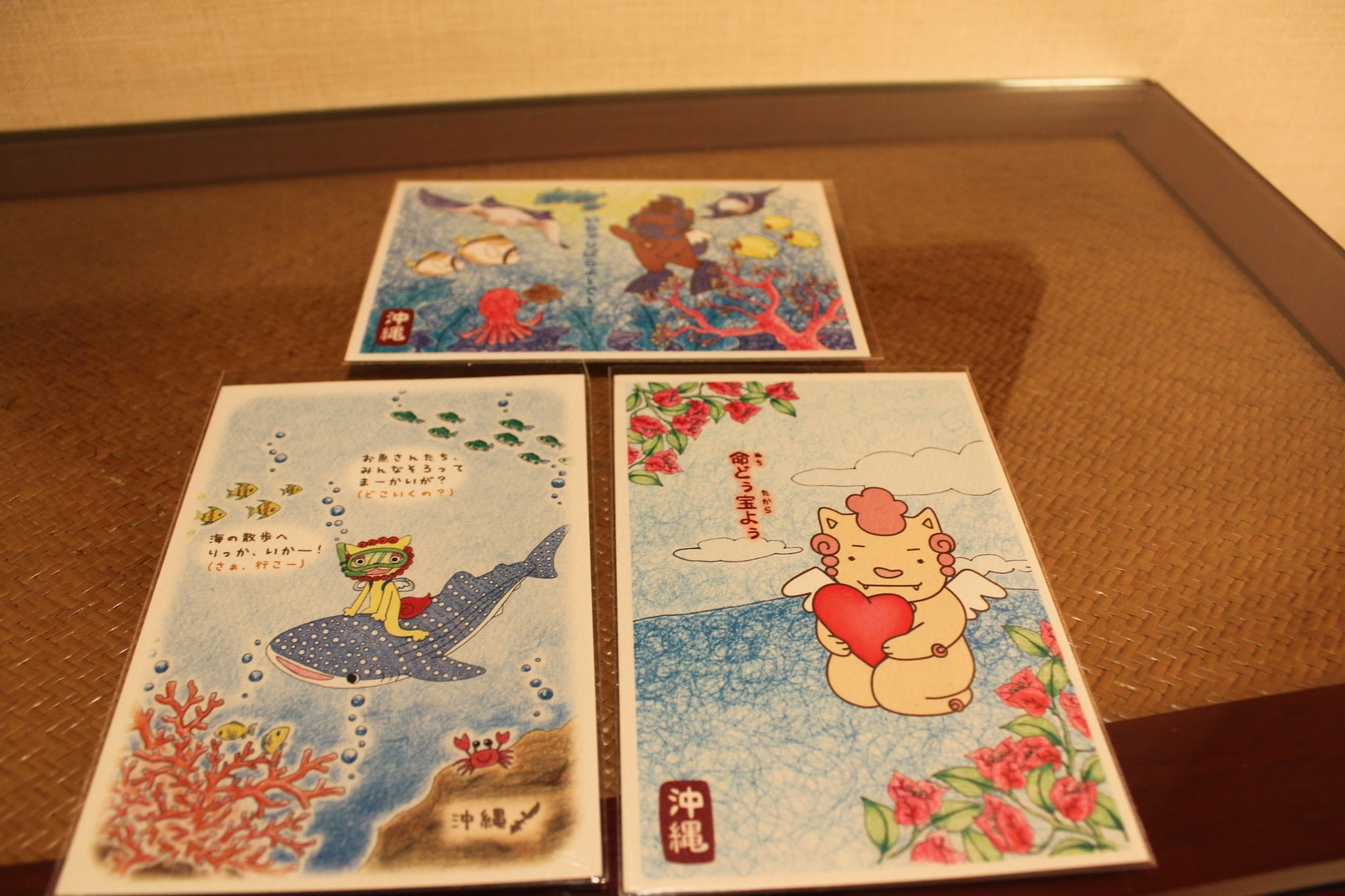The image showcases three vibrant children's illustrations, neatly arranged on a brown wooden tray. The top illustration features an ocean scene set against a white background with splashes of blue and dark blue hues. It depicts a lively underwater world with a yellow fish, a red octopus, and several other colorful marine creatures. Intriguingly, there appears to be a character engaged in scuba diving.

The illustration below, situated on the left, also portrays an underwater adventure. It focuses on a small, yellow creature wearing a face mask, joyfully riding a blue whale adorned with white spots. The scene is further enriched with seaweed in the bottom left corner, a little red crab, and various green and yellow fish swimming around. The background is a deep, soothing blue, and there is visible text in what seems to be an Asian language.

The final illustration, located to the right, presents a whimsical, flesh-colored cat holding a large heart while sitting on a blue ground. The backdrop features a blue and white sky. The scene is accentuated with Asian characters in red, along with roses positioned in the upper left and bottom right corners, adding a touch of floral charm to the illustration.